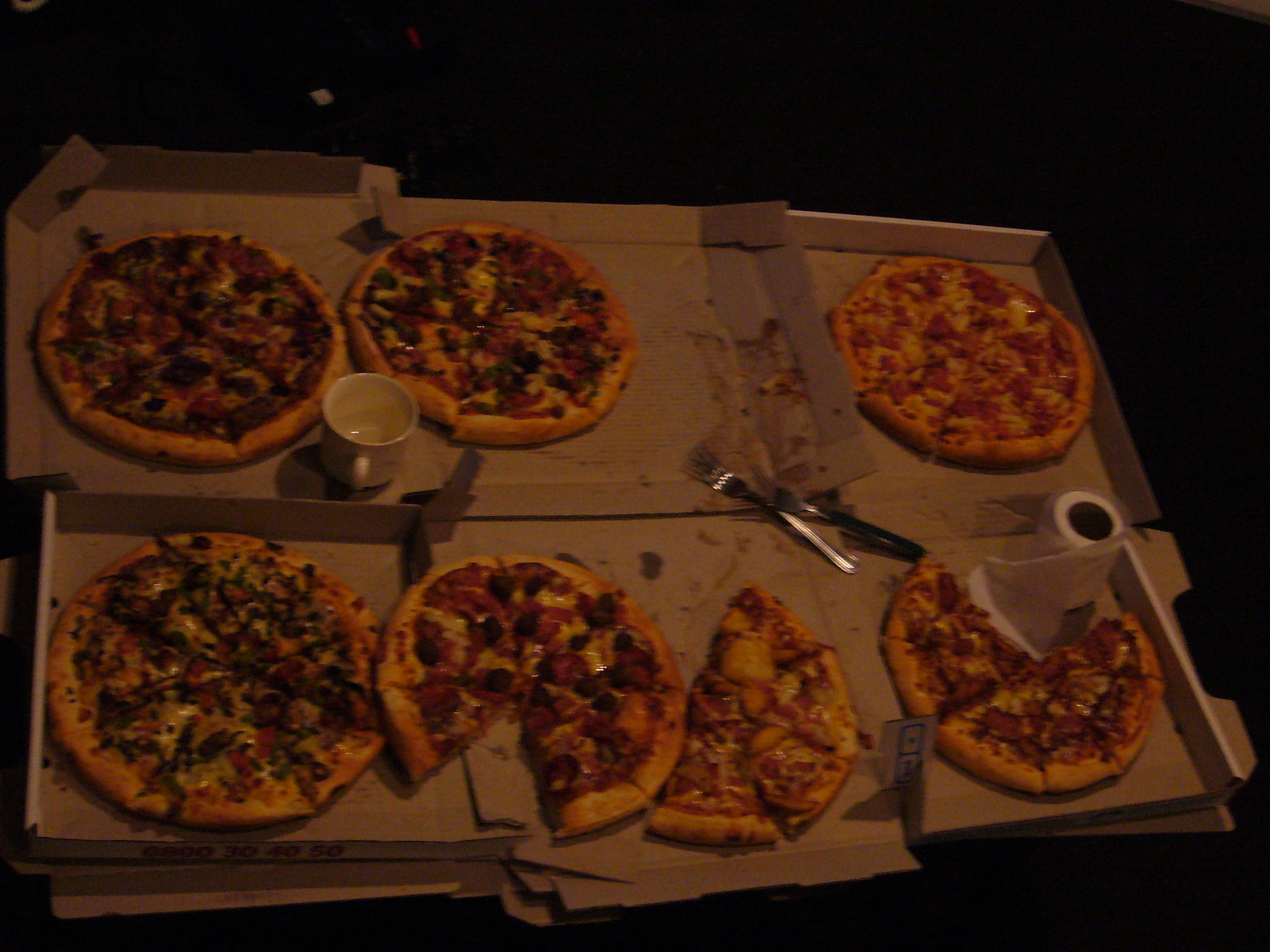This dimly lit and blurry photograph depicts seven pizzas arranged in opened pizza boxes forming a rectangle against a dark background. Among the pizzas, three remain intact, showcasing toppings that likely include dark-colored ingredients such as olives and meats, alongside what might be pineapple and green vegetables. Four pizzas have been partially consumed, with missing slices creating an untidy display. Centered among the pizzas are used silver utensils—two forks and a butter knife—amid smudges of spilled grease. A white, empty coffee mug sits between two of the untouched pizzas, while on the right, where some slices are missing, a roll of toilet paper is conspicuously placed. Text in blue and red colors is faintly visible on one of the pizza boxes, adding to the chaotic scene.